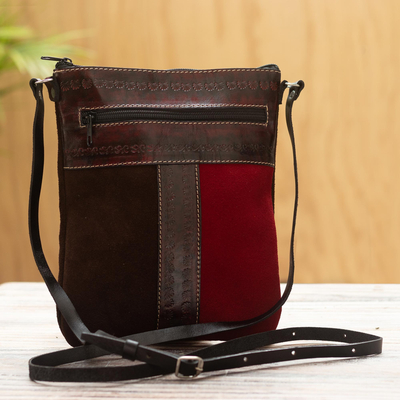This photograph showcases a stylish, compact satchel or handbag, set on a white table, possibly marble, against a warm orange-yellow wooden wall backdrop with a green plant leaf entering from the left. The satchel features a rich, dark red-brown leather exterior with intricate stitch designs and pressed patterns. Central to its design are two zippers: one at the top providing access to the main compartment, and another along a leather strip in the middle forming an outer pocket. The bag's long, adjustable leather strap, equipped with metal buckles, offers versatile carrying options—either on one shoulder or as a crossbody. The bottom section of the bag is adorned with distinct segments of red and blue fabric, adding a vibrant contrast that hints at a possible Tommy Hilfiger design, though the materials might also include velveteen for a tactile finish. Though small, this bag is practical, ideal for essentials like a wallet and lipstick.